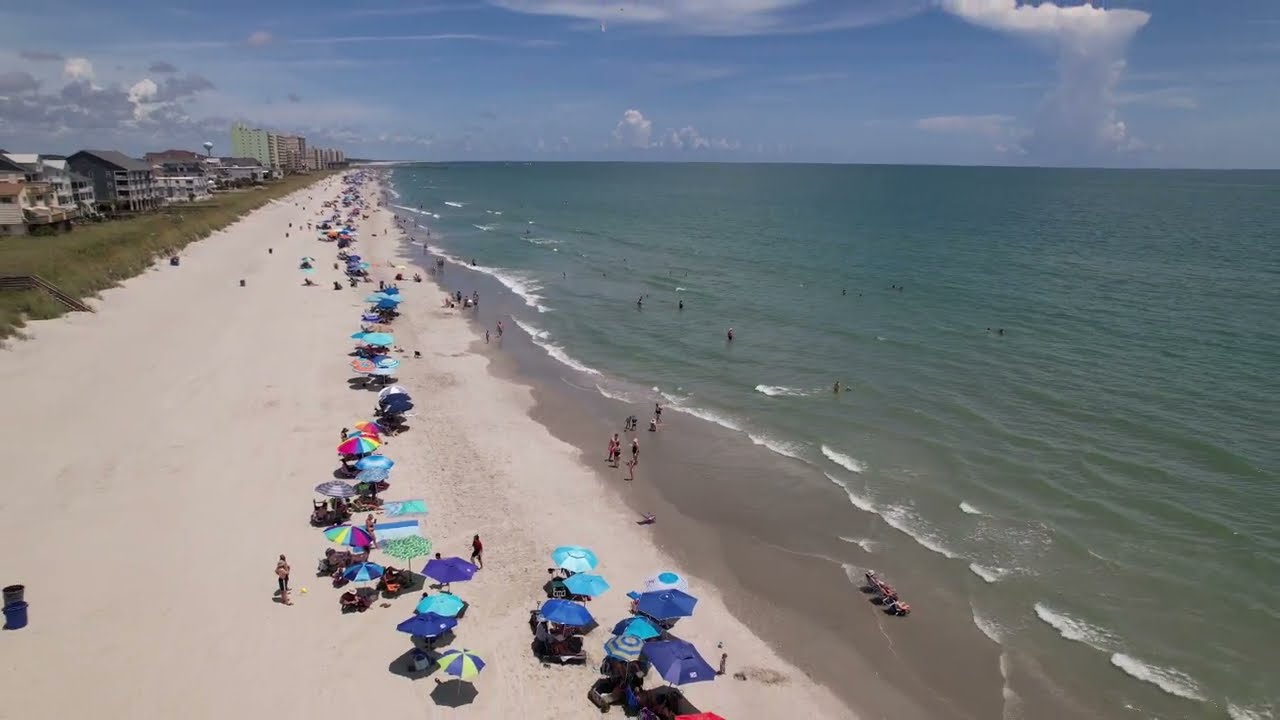The image captures a bustling beach scene where the sandy shoreline stretches into the horizon, situated on the left-hand side of the photo, and meets the blue-green water on the right. Numerous vibrant umbrellas dot the beach, primarily in shades of blue, with splashes of rainbow colors, bright neon blue, yellow, pink, and purple. The water, slightly choppy with whitecaps, hosts several people enjoying the waves, while others stroll along the shore or relax under their umbrellas, creating a lively yet not overly crowded atmosphere.

In the background, a green embankment transitions from the sandy beach to a series of buildings, possibly hotels or homes, that overlook the waterfront. The sky above is a striking blue adorned with large, thick white clouds, adding to the pleasant and inviting environment of the day. The image encompasses a wide array of colors including blues, tans, greens, and specks of various bright hues, all contributing to the vibrant and dynamic scene.